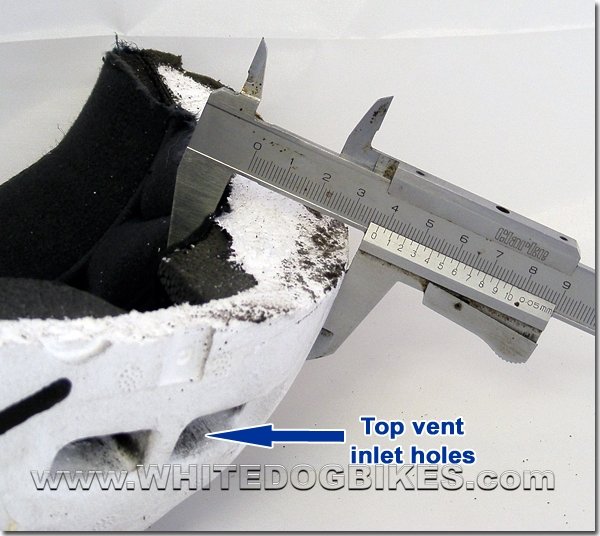The image displays an intricately detailed view of a segment of a bike helmet. The helmet, predominantly white with a black interior, features a texture that resembles snow or chalk. Positioned on its top side, possibly upside down, the helmet part is under measure by a silver caliper, recording its width at approximately three and a half inches. Prominently, a blue arrow with white borders points to one of the square vent openings on the helmet, labeled "top vent inlet holes" in blue text. The background is a plain white surface, accentuating the outlined elements. At the bottom, the website "www.whitedogbikes.com" is displayed in clear, shadowed text.